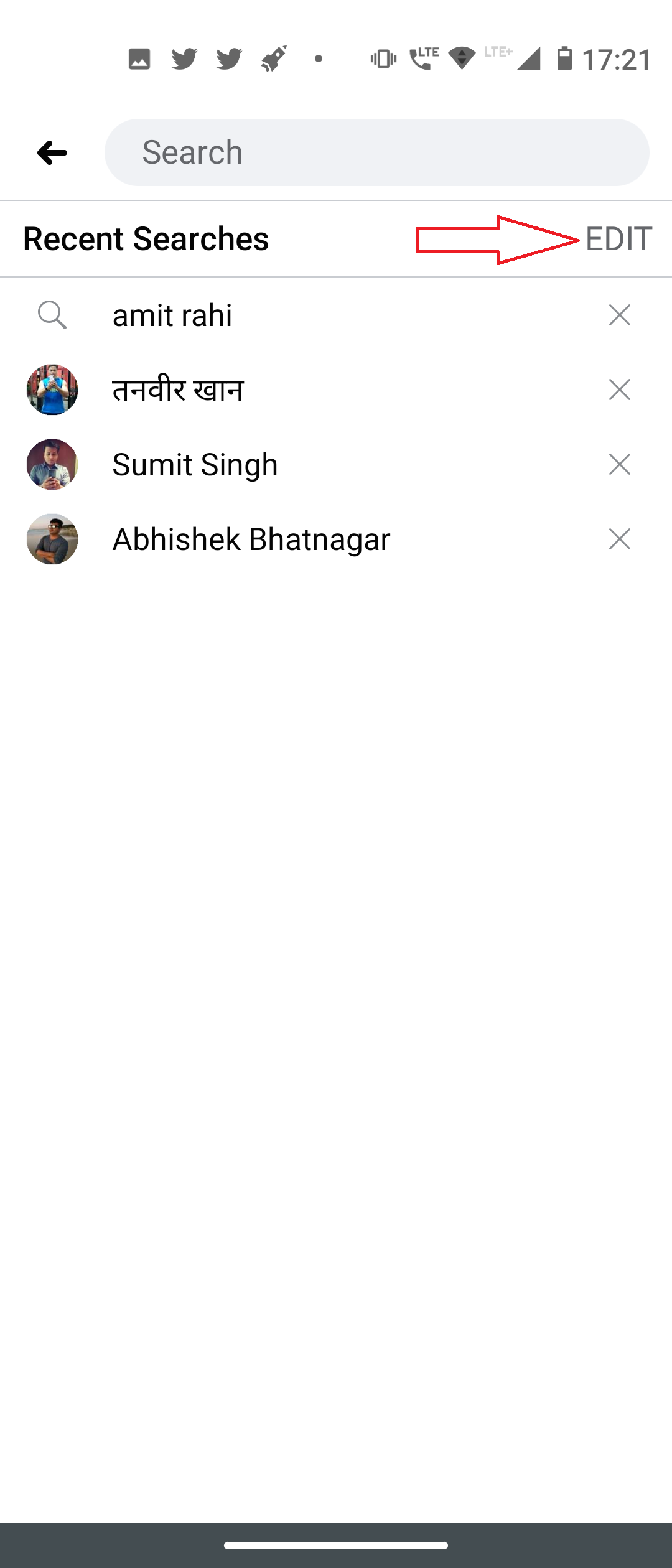A high-resolution image of a smartphone screen showing a Twitter interface. The phone is in vibrate mode, as indicated by the icon on the status bar, which also displays signal bars, Wi-Fi connectivity, battery level at 17:21, and a search bar. The search bar is grey and features a black left arrow, the text "Recent searches," and an "Edit" option in grey at the right end.

Below this section, a white arrow with a red outline points towards the search bar, with the text "AMIT RAHI" underneath it. To the right of this text, beneath the "Edit" option, is an "X" button adjacent to some text written in an unknown language. This pattern repeats below with the names "SUMMIT SINGH" and "ABHISHEK BHATNAGAR," each accompanied by an "X" button on the right.

The lower section of the screen features a significant expanse of white space and concludes with a black band at the bottom, marked by a central white line. The image appears to serve educational purposes, with the prominent arrow likely used to guide or instruct the viewer.